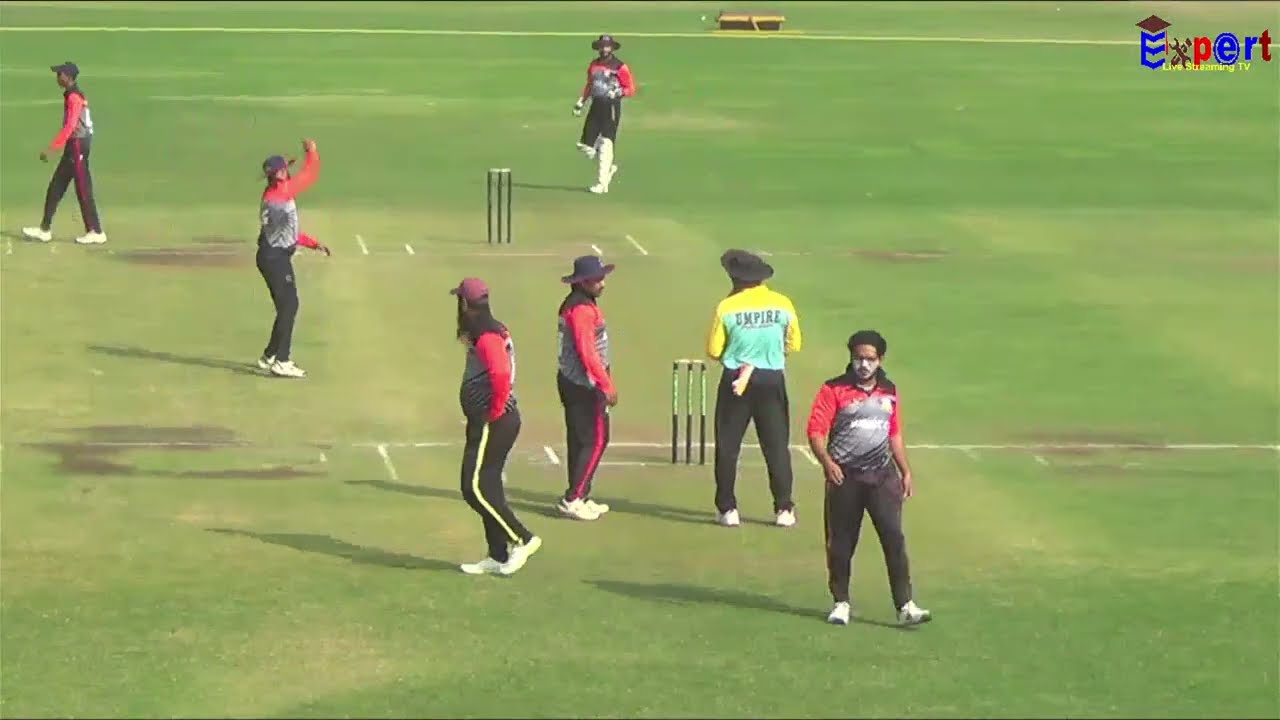The image captures a group of seven men on a grassy field, engaged in what appears to be a cricket match under a bright, sunny sky. Six of these men are outfitted in uniforms consisting of red shirts with silver details, black pants, and hats, while a seventh individual, likely the umpire, stands apart in a blue and yellow shirt with "UMPIRE" written on the back, also wearing black pants. The field is marked with white lines and rectangular boundaries typical of a cricket pitch. In the upper right corner of the image, a logo reads "Expert Live Streaming TV," indicating that the event is being broadcast live. A stand holding what looks like cricket bats adds to the authenticity of the setting. All participants are in position, seemingly preparing for the start of play. The scene suggests a sense of anticipation and readiness among the players.